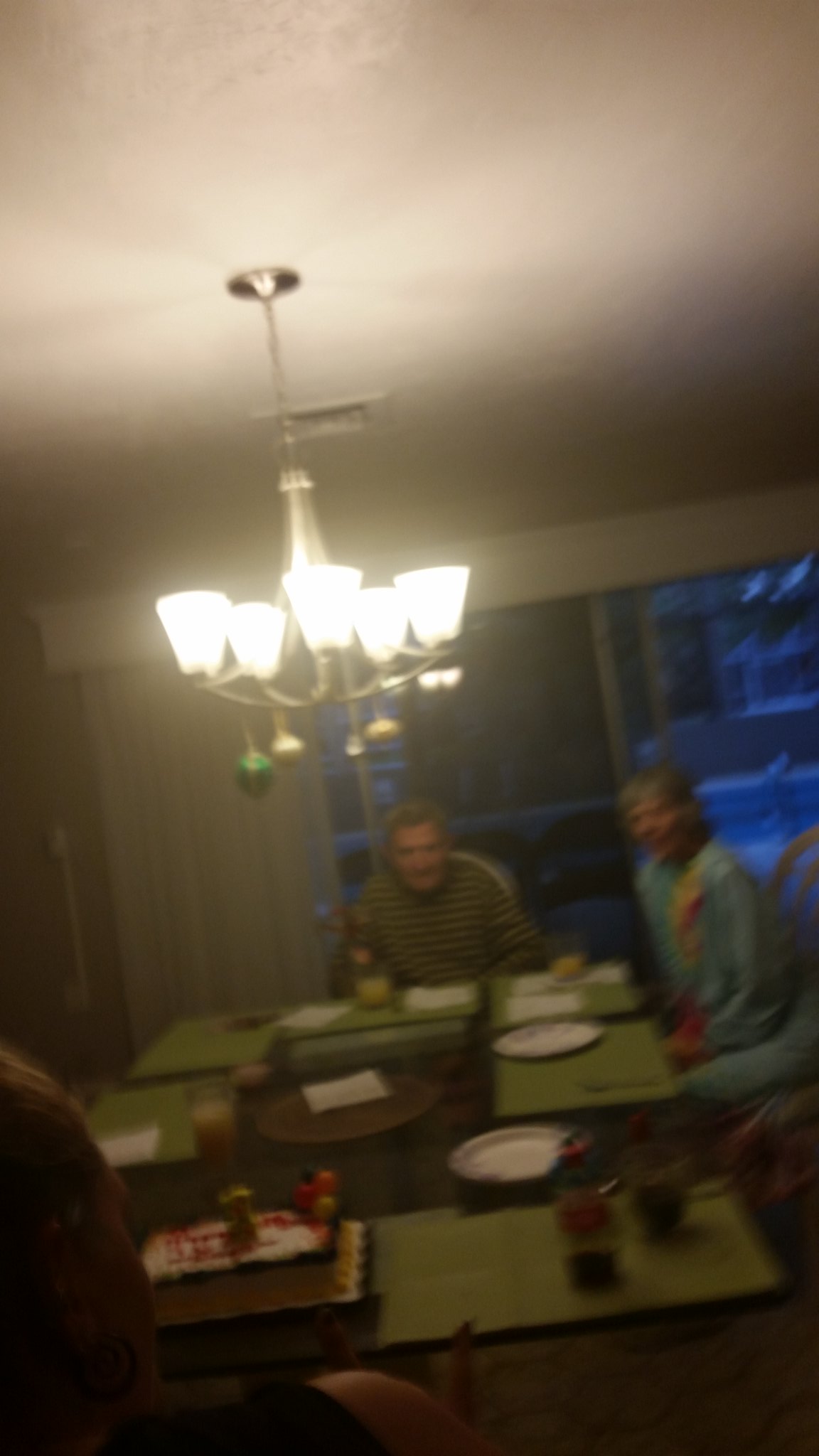In this slightly blurry photograph, a family is gathered around a large rectangular dining table in a cozy living room. The backdrop reveals a homey atmosphere with a large floor-to-ceiling window adorned by a white, floor-length drape. The drape is partially drawn open, with much of it gathered neatly along the left-third of the window. 

At the head of the table sits an elderly gentleman, whose presence is accentuated by a bottle of alcohol placed in front of him. The dining table is meticulously set with placemats for six, suggesting a family meal in progress or about to begin. On the right side of the table, an elderly woman with short gray hair dressed in a light blue top is visible, adding to the family gathering's warmth.

In the foreground, the perspective is over the shoulder of a woman with blonde hair, who is wearing a black sleeveless top. She appears to be captivated by a birthday cake placed on the table. The cake itself is white, trimmed with a blue border, and features a red inscription that is not fully legible. Notable decorations include a plastic bunch of balloons positioned at the cake's corner and a number candle standing prominently on top, signifying the celebration of someone's special day. Several plates are visible around the cake, ready for what promises to be a joyous occasion.